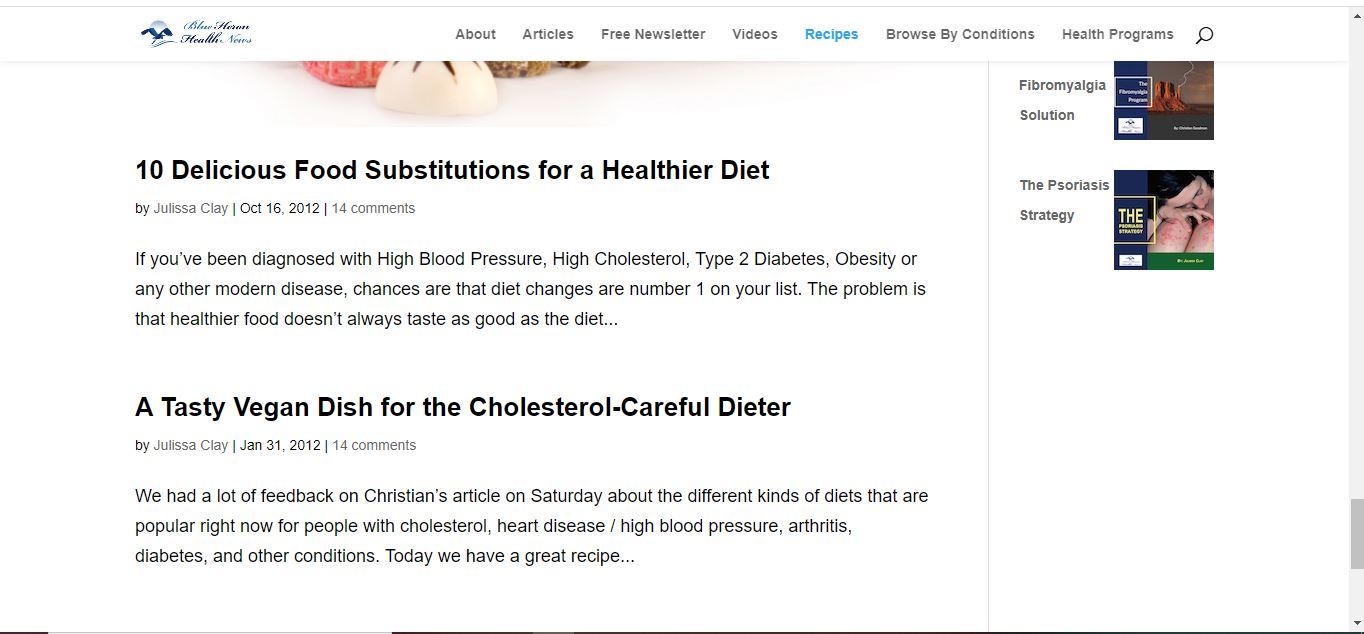This screenshot depicts a web page from a health-related website. On the right side of the screen, a progress bar indicates that the viewer is near the bottom of the site. The top section of the page is faintly visible, displaying an eagle logo and some cursive text, followed by menu headings such as "About," "Articles," "Free Newsletter," "Videos," "Recipes," "Browse by Conditions," and "Health Programs."

The "Recipes" section has been selected, likely causing the page to scroll down to the relevant content section via bookmarks. Two recipe articles are prominently featured. The first article is titled "10 Delicious Food Substitutions for a Healthier Diet," aimed at individuals diagnosed with conditions like high blood pressure, high cholesterol, type 2 diabetes, or obesity. The introductory text suggests that dietary changes are critical for managing these conditions, but acknowledges the challenge of finding healthy food that tastes good, ending with an ellipsis.

The second article is titled "A Tasty Vegan Dish for the Cholesterol-Careful Dieter." It also includes a brief introductory blurb similar in style to the first article, presumably discussing the benefits of vegan recipes for those monitoring their cholesterol levels.

The screenshot captures these elements but lacks visibility of the authors' names due to the page design or image resolution.